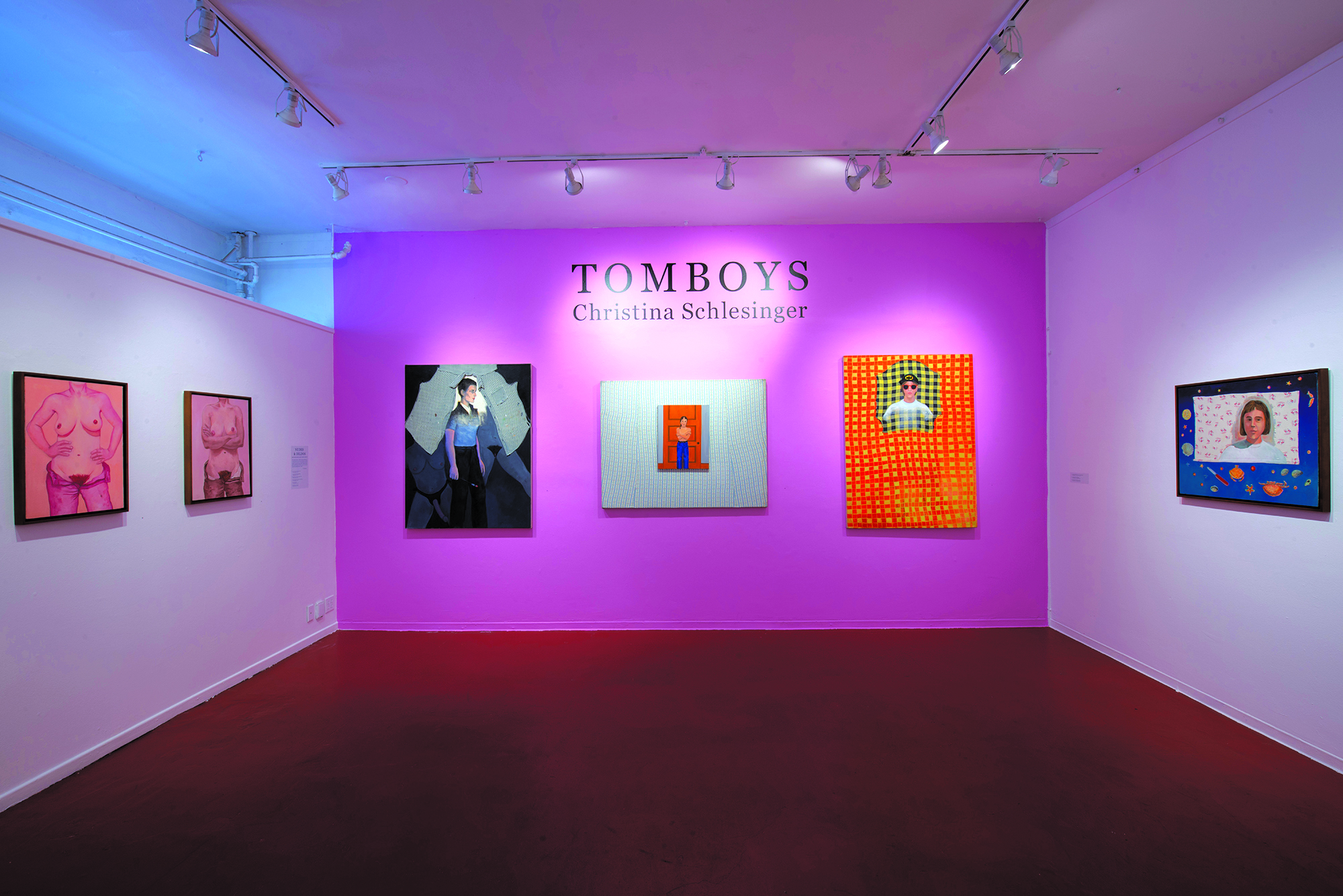The image depicts an art gallery room with a distinct aesthetic. The primary focus is a vivid purple back wall featuring the text "Tomboys, Christina Schlesinger, S-C-H-L-E-S-I-N-G-E-R" prominently displayed. The room is bathed in light from rows of spotlights mounted on metal rods across the ceiling, illuminating the artworks on display. The gallery's ceiling and side walls are white, while the floor contrasts sharply with a bright burgundy red hue.

The back wall is adorned with three primary paintings. On the far left, there are nude paintings of women that prominently display their forms. The central artwork features a red door, capturing attention with its bold color. The painting on the right showcases a person against a plaid pattern. Additionally, a painting on this wall depicts a man dressed in black pants, surrounded by green.

The detailed and varied artwork highlights themes of human form and identity, with a recurring focus on both male and female figures. The presentation of these pieces against the vibrant and contrasting colors of the gallery accents the boldness of Christina Schlesinger's exhibit, contributing to a compelling and provocative artistic experience.